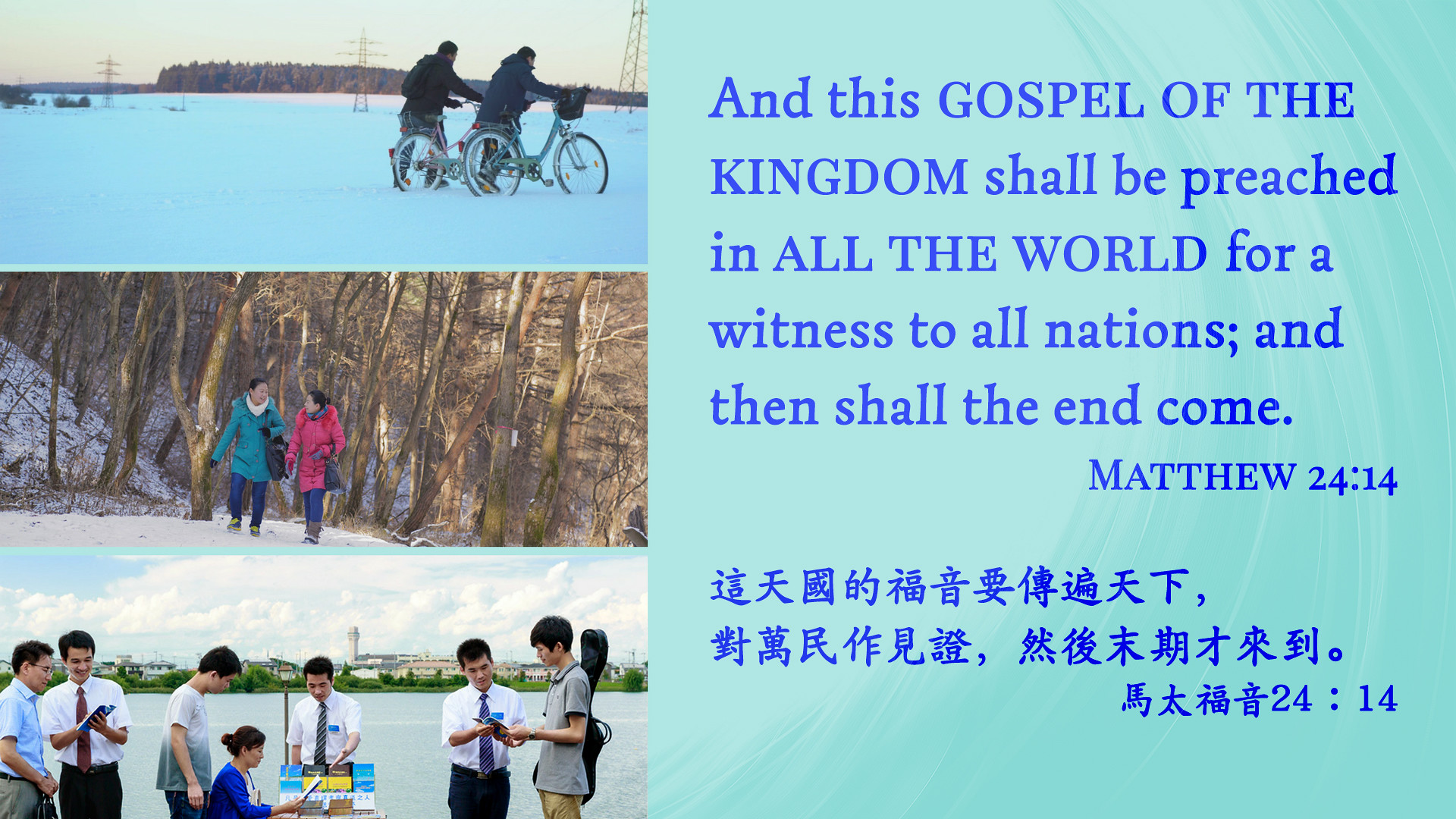The image is divided into two sections. On the right half, a turquoise background features a quote in blue text: "And this gospel of the kingdom shall be preached in all the world for a witness to all nations, and then shall the end come. Matthew 24, 14." Below the quote is an apparent translation into Chinese characters. The left half of the image consists of three vertically stacked photographs. The top photo shows two men pushing bicycles through a snowy field. The middle photo depicts two women dressed in winter clothing walking along a snowy path, with trees visible in the background. The bottom photo captures a group of young people, including men and one woman, gathered around the edge of a lake. They appear to be exchanging information and are looking into books or pamphlets.